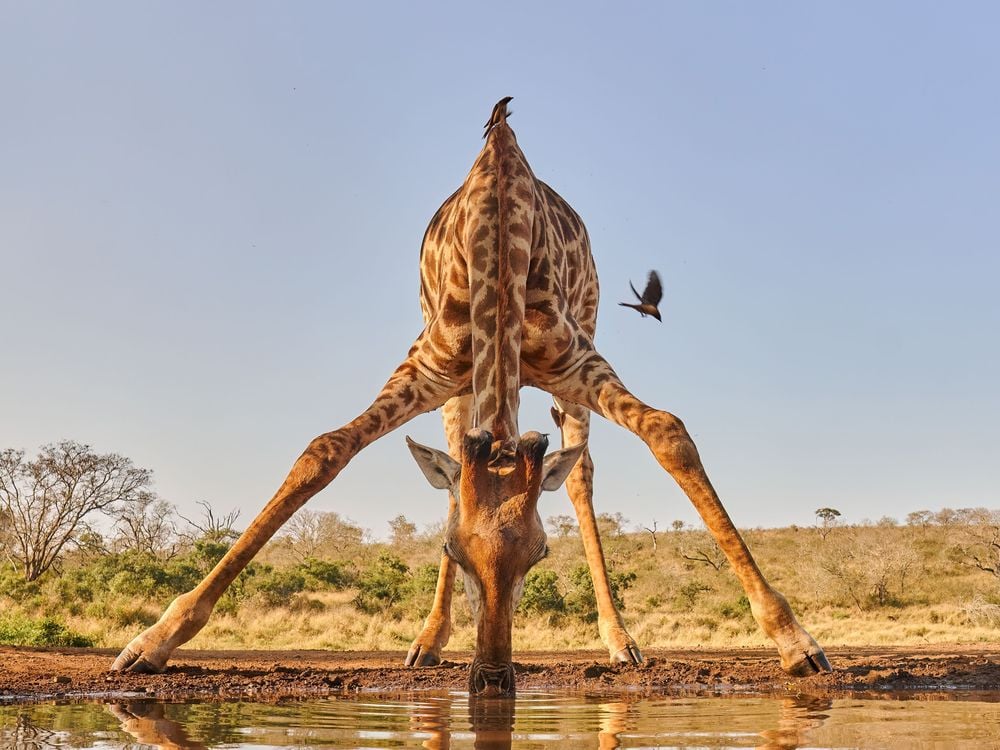In this detailed close-up image, a giraffe with yellow fur and darker orange-brown spots is bending down to drink from a small, muddy pond. To accomplish this, the giraffe has splayed its front legs wide apart while keeping its back legs straight, making its posture quite comical. Its ears poke out to the sides, and its nose or snout is immersed in the water. The giraffe's head is adorned with two small antlers, indicating it could possibly be a juvenile. Nearby, a small black bird is captured in flight, positioned to the giraffe's right. The setting seems to be an African savanna, with a mix of yellow grass, green shrubbery, and brown shrubs visible in the background. A tree with sparse leaves stands in the very left-hand corner of the picture, and the scene is bathed in the light of a clear blue sky.